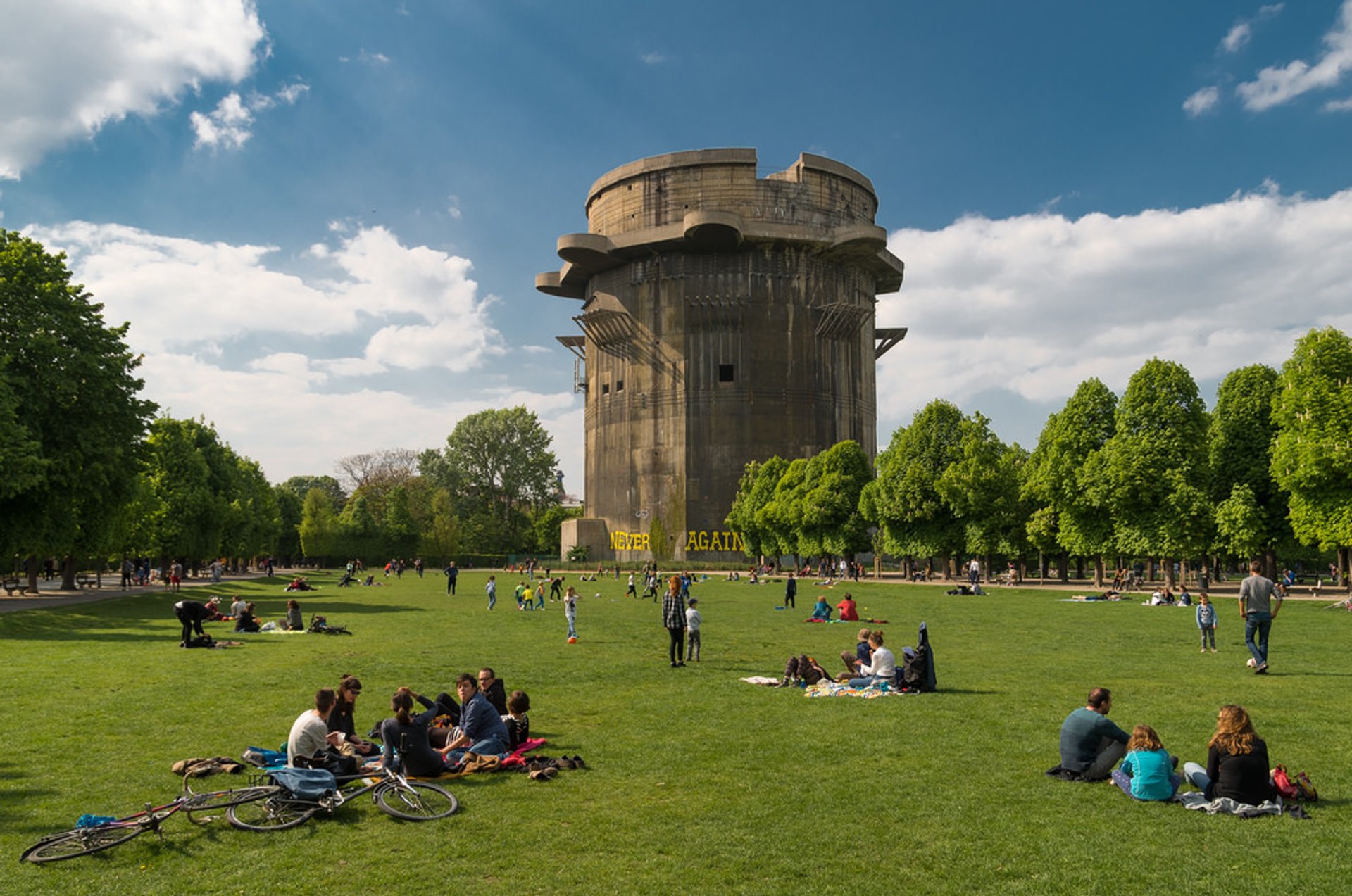The photograph depicts a park on a sunny day with a mostly blue sky dotted with wispy clouds. At the center of the image, there is a large, dark brown, cylindrical tower, resembling a missile silo, with a rim on top. Painted in large yellow letters at the base of the tower are the words "NEVER AGAIN." Elm trees surround the site, and a broad, lush green lawn extends across the park. Scattered throughout the lawn are about fifty people engaged in various activities typical of a summer day — picnicking, playing ball, chatting, and simply relaxing. Bicycles lie on the grass, and there is one person in the foreground, sitting on a towel or blanket, looking directly at the camera amidst a group of friends. The vibrant, communal atmosphere contrasts with the stark message on the silo, creating a striking scene of serenity and solemn remembrance.